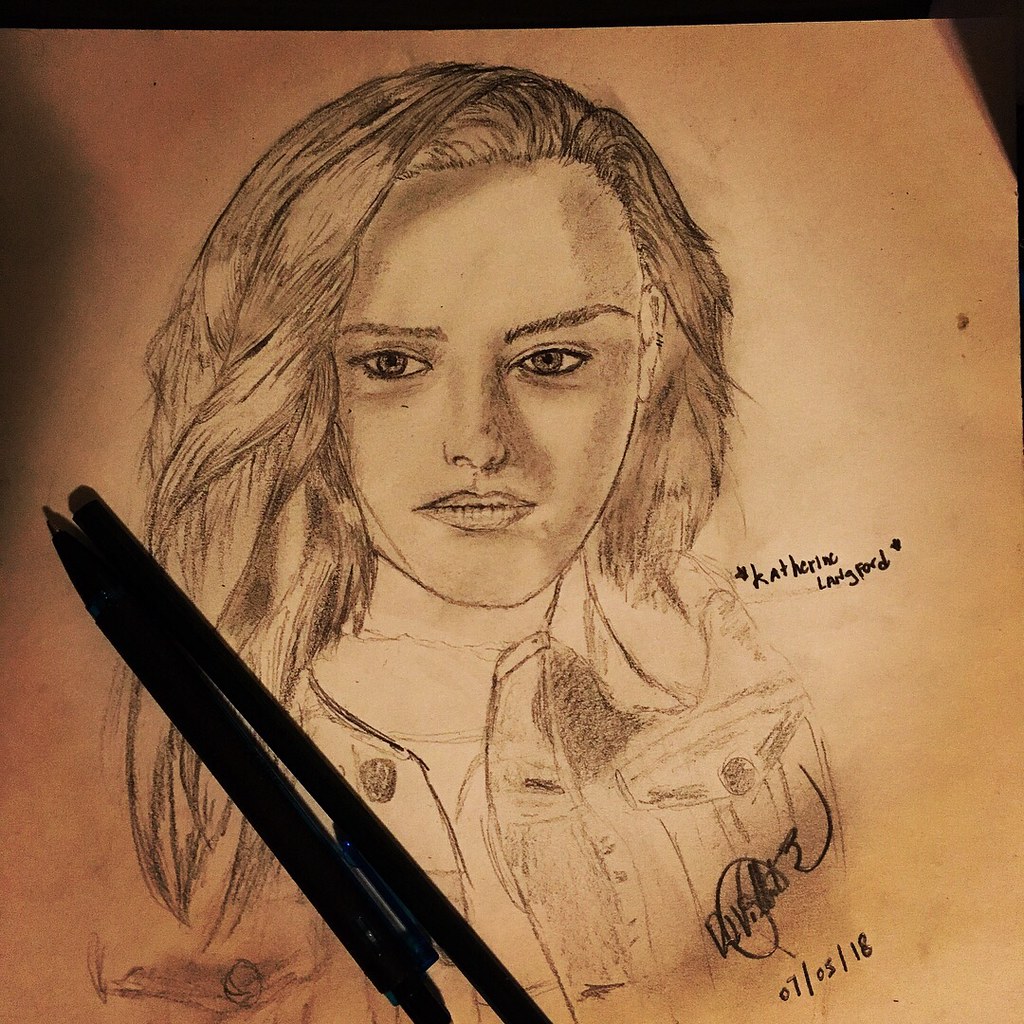The photograph showcases a dimly lit image of a sketch on a piece of paper that appears to be beige or white but looks tan due to the lighting. The paper is against a black border at the top and top-right corner. Two dark pens or pencils lie diagonally crossing the lower left-hand corner, casting subtle shadows. The sketch itself is a finely detailed portrait of a young woman with long, wavy hair. She has a serious expression, with thin, angled eyebrows and a full, closed mouth. The drawing captures her wearing an unbuttoned jacket over a shirt. The shadowing around her nose and eyes enhances the depth, with bright white highlights around her eyes. To the right of the woman, the name "Catherine Langford" is written, while the lower right-hand corner bears a signature and the date "07/05/18."